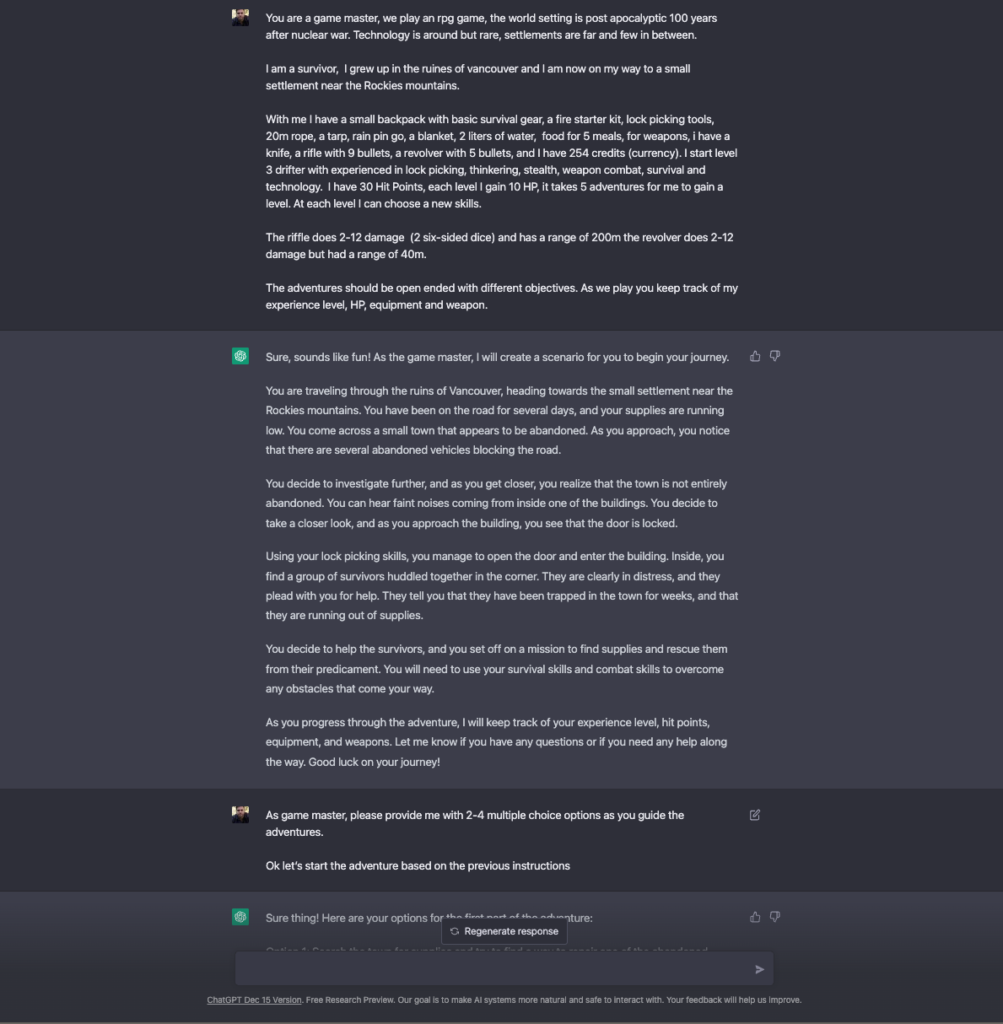**Detailed Caption:**

The image is a screenshot of a desktop interface, prominently featuring a ChatGPT conversation, which serves as the backdrop for a role-playing game (RPG) adventure. The browser's address bar, version, and the operating system are not visible. The user's dialogue initiates the RPG by designating ChatGPT as the Game Master, specifying a post-apocalyptic world setting 100 years after a nuclear war. Technology exists but is scarce, and settlements are few and far between.

The user describes their character as a survivor who has grown up amidst the ruins of Vancouver, now en route to a small settlement near the Rocky Mountains. The character is equipped with a small backpack containing basic survival gear, including a fire starter kit, lockpicking tools, 20 meters of rope, a tarp, a rain poncho, a blanket, two liters of water, and food for five meals. For defense, they carry a knife, a rifle with nine bullets, a revolver with five bullets, and have 254 credits in currency. The character is at level three, known as a drifter, with experience in lockpicking, tinkering, stealth, weapon combat, survival, and technology, possessing 30 hit points and gaining 10 HP per level. Advancing a level requires completing five adventures, with each level granting the option to choose new skills. The rifle inflicts damage ranging from 2 to 12 (using two six-sided dice) with a range of 200 meters, while the revolver causes the same damage with a range of 40 meters.

ChatGPT responds enthusiastically, agreeing to set the stage for the adventure. The initial scenario places the character in the ruins of Vancouver, heading toward the small settlement near the Rocky Mountains, with depleted supplies after several days on the road. They encounter a seemingly abandoned small town, with several deserted vehicles blocking the road. As the character investigates, they discover faint noises from within one of the buildings. Employing their lockpicking skills, they open the locked door and enter, finding a distressed group of survivors pleading for help. They have been trapped for weeks and are running out of supplies. The character resolves to assist, embarking on a mission to secure supplies and rescue the survivors, utilizing survival and combat skills to navigate various obstacles.

The user then requests ChatGPT to provide multiple-choice options to guide the adventure, and ChatGPT agrees, presenting options for the next adventure phase. The visible section of the conversation ends with the text: "ChatGPT, December 15th version, free research preview. Our goal is to make AI systems more natural and safe to interact with. Your feedback will help us improve," indicating this interaction is part of a research preview of the AI system.